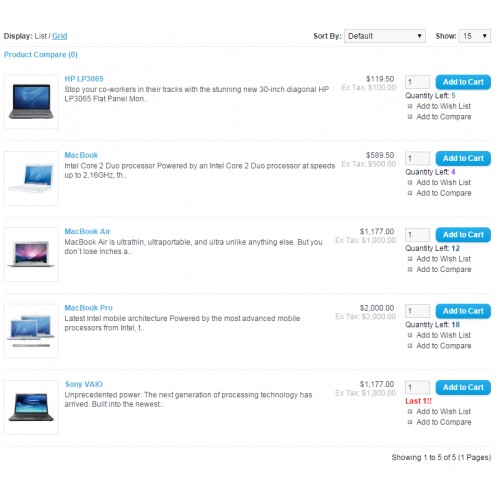Screenshot of an online product page showcasing various electronics with detailed information:

In this screenshot, a list and grid view option is presented at the top, allowing users to display items either in a list or grid format. The page features a "Product Compare" option and sorting capabilities with a default setting. Users can choose to display 15 products per page.

Highlighted products include:

1. **30-Inch HP Flat Panel Monitor (HPLP3065)**:
   - Description: "Stop your co-workers in their tracks with the stunning new 30-inch diagonal HP flat panel monitor."
   - Price: $119.50
   - Quantity Left: 5
   - Availability: Add to cart option available

2. **MacBook**:
   - Price: $589.50
   - Quantity Left: 12
   - Availability: Add to cart option available

3. **MacBook Air**:
   - Price: $1,177.00
   - Quantity Left: 12
   - Availability: Add to cart option available

4. **MacBook Pro**:
   - Price: $2,000.00
   - Quantity Left: 18
   - Availability: Add to cart option available

5. **Sony VAIO**:
   - Price: $1,777.00
   - Note: Last one available
   - Quantity Left: 1
   - Availability: Add to cart option available

The text detailing these products is primarily in black, with the "last one" note for the Sony VAIO and the quantity left for the MacBook (4) rendered in a reddish hue. The pagination at the bottom indicates that this is showing items 1 to 5 of 5, across a single page.